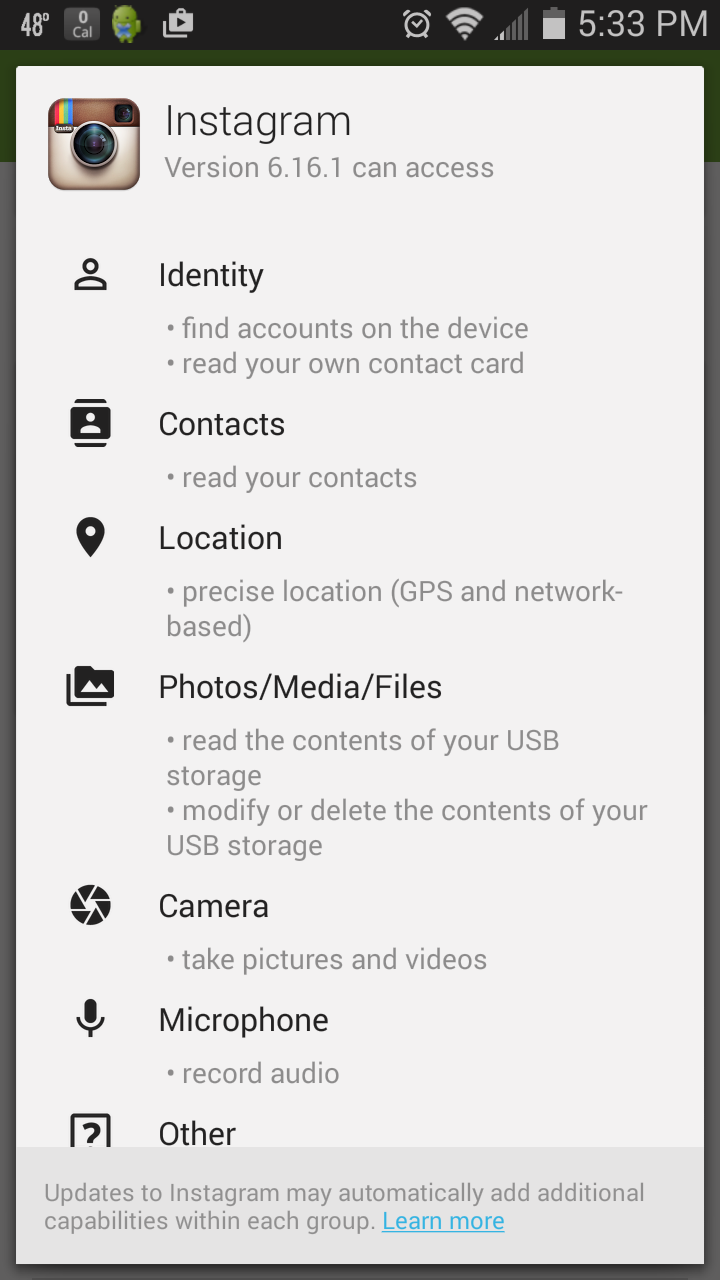The image showcases a smartphone screen displaying a permissions request for Instagram version 6.16.1. The top of the screen shows key status indicators, including a temperature reading of 48 degrees on the left, a zero overlaid with a cow icon, an alarm symbol, Wi-Fi strength, cellular signal bars, and a battery icon that is mostly charged. The time is displayed as 5:33 PM.

The background is predominantly black with a prominent white rectangle overlay, within which the permission details are listed in black font on a grayish-white background. The heading reads "Instagram version 6.16.1" followed by an extensive list of permissions the app requests. These permissions include access to identity information, the ability to find accounts on the device, read the user's contact card and contacts, access precise location based on GPS and network data, read and modify the contents of USB storage, take pictures and videos, record audio, and potentially gain new capabilities through updates.

Additionally, there is a "Learn more" link highlighted in blue and underlined. The permissions request raises concerns about privacy due to the extensive access required by the app. There is also a small icon in the interface that appears to be a stylized camera with the word "Insta" on it, colored in light and dark brown hues with various additional colors.